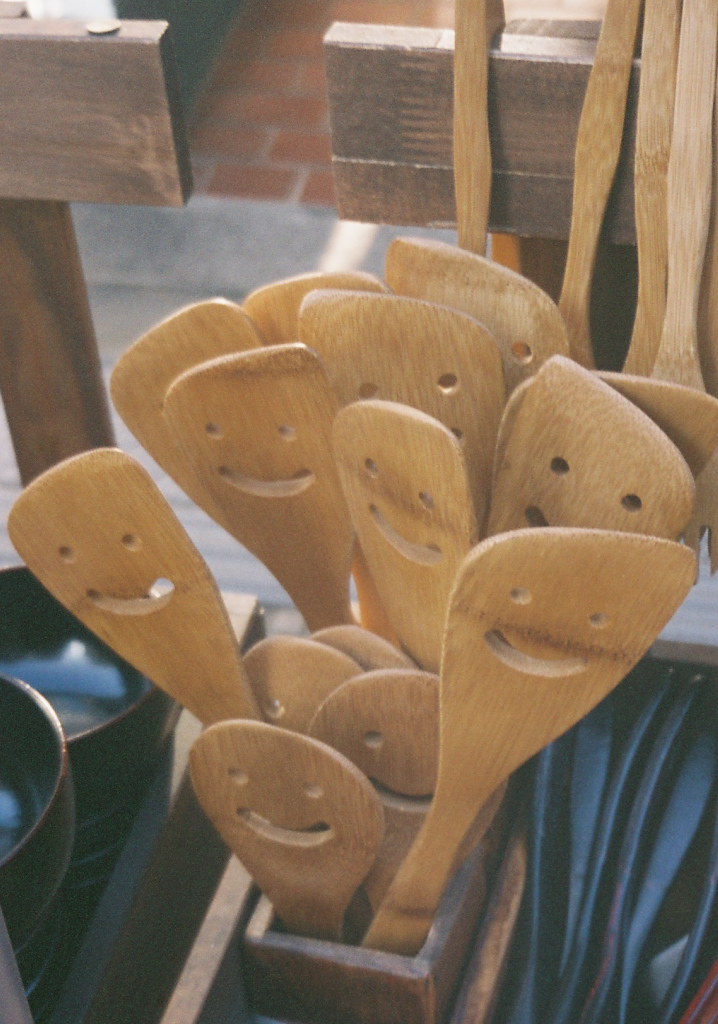A close-up exterior photo captures an assortment of wooden kitchen utensils, prominently featuring wooden spoons and spatulas with slotted, smiley face designs. These utensils, of varying heights and shapes—some with round ends and others with flat or angled ends—are neatly displayed in a rectangular wooden container. Each utensil has perforations that form a cheerful face with two small circular eyes and a curved, upward-turned mouth. In the background, an assortment of wooden utensils hangs vertically, adding rustic charm to the scene. To the left, a wooden crate holds a stack of black bowls, while a crate on the right contains flatware. The backdrop includes a gray concrete surface and brown brick flooring, enhancing the country-style ambiance of the setting.